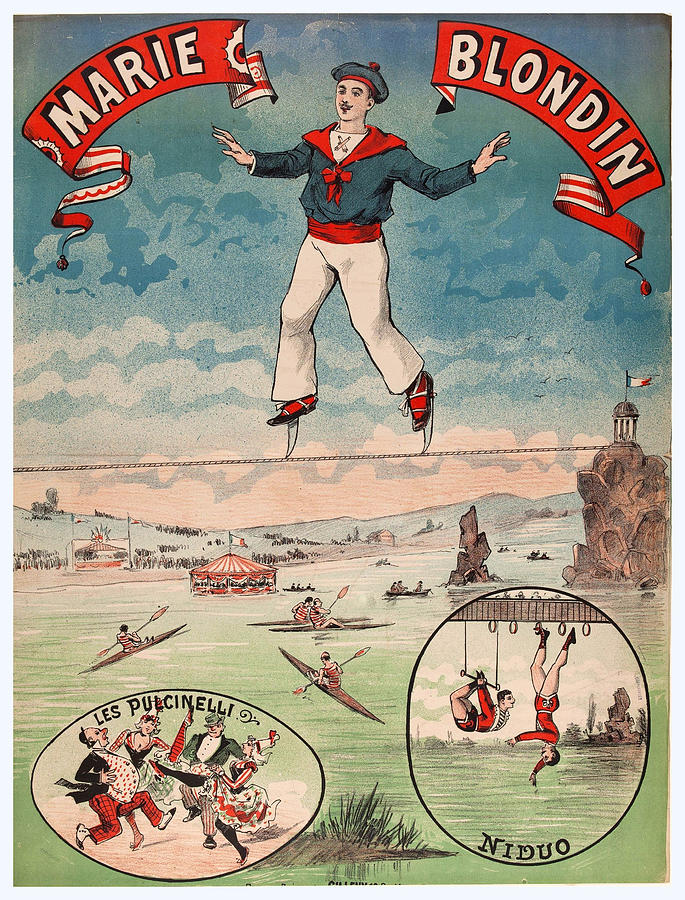This vintage circus poster features a striking illustration of a French tightrope walker, identified by the large red banners as Marie Blondin. The banners at the top left and right proclaim "Marie" and "Blondin" respectively, adorned with intricate designs and ribbon-like tails. At the center, the tightrope walker, distinguished by his beret, mustache, and traditional outfit consisting of a navy top with red accents, white pants, and stiletto-like tightrope shoes, is suspended above a body of water. Below him, numerous kayakers navigate the waters, with a circus tent seemingly afloat. In the background, another circus tent is visible, surrounded by crowds on the hillsides. The poster also includes scenes of circus performers: on the bottom left, a group of dancers labeled "Le Pulcinelli," and on the bottom right, acrobats labeled "Niduo," hanging from a trapeze and rings. The image, with its retro and detailed artistic style, captures the grandeur and festive spirit of the circus.